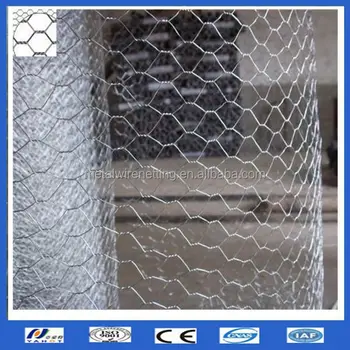The image is a detailed close-up of partially rolled-out chicken wire, captured within a white frame bordered by a blue frame. The foreground prominently features the chicken wire, which spans almost the entire width of the image, with a spool visible on the left side. A small white sticker on the wire reads "Wiredheading.en.alibaba.com." The backdrop reveals a warehouse-like environment, characterized by a half white, half brown wall, a brown floor, and indistinct black items that appear to be filing cabinets or other black products. The blue border at the bottom is elongated and contains five somewhat stretched logos, among them "CE" and "IAF" on the far right, likely indicating various company certifications or affiliations, though the remaining logos are hard to decipher due to image quality constraints. This intricately framed scene suggests a construction or contracting site.